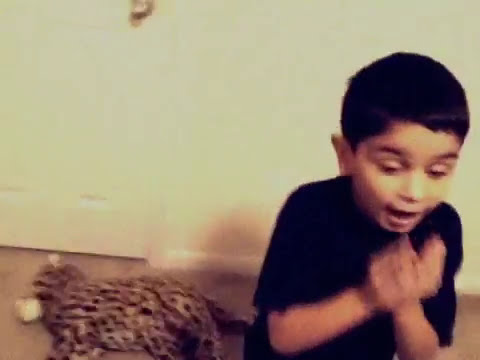A young boy with short dark brown or black hair, dressed in a black t-shirt, appears on the right side of the image. His expression is one of shock or surprise, with his mouth slightly open, eyebrows raised, and eyes widened. His hands are crossed over each other, forming a subtle X shape in front of him, and his posture suggests he's gasping or reacting to something. The lighting highlights his nose prominently, indicating a strong light source nearby. To his left, near the bottom of the image, is a dark-colored cat-like figure that could be a plush toy or a stuffed animal, resembling a cheetah or a panther, with golden tan skin and black dots. The floor beneath him is a light tan wood, and behind him is a plain white wall. On the far left, a white door with a yellow handle interrupts the wall's expanse. The image quality is quite low, with muted colors and noticeable blur, making finer details indistinct.